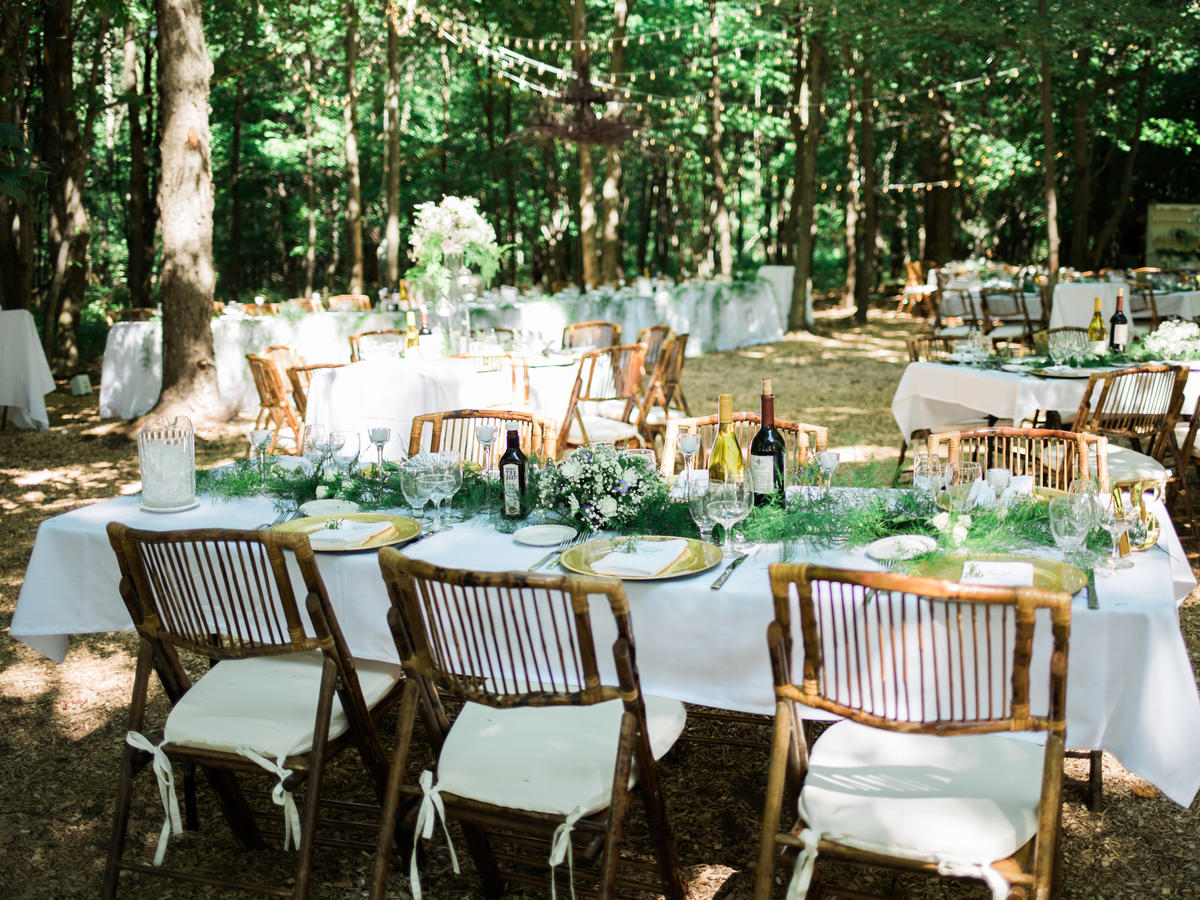The image showcases a meticulously arranged outdoor wedding reception set amidst a garden filled with tall, green-leaved trees with brown trunks. The venue embraces a rustic and natural ambiance, adorned with light garlands hanging gracefully from the trees, illuminating the area with a warm, festive glow. A plethora of rectangular and some round tables, covered in elegant white tablecloths, are arranged throughout the area. The tables feature white cushioned, rustic brown wooden chairs that add to the earthy charm. 

Each table is beautifully decorated with a garland of greenery running across its center along with white floral arrangements, embodying the white and green wedding theme. Golden plates set at every place setting are complemented by neatly folded white napkins, silver cutlery, and a trio of glasses - a water glass, red wine glass, and white wine glass. White votive candles in tall stemmed glass holders and bottles of red and white wine enhance the celebratory feel. Some tables also feature additional decorative touches like flower vases.

Prominent in the arrangement is a large banquet table situated in a clearing, flanked by trees on either end, distinguishing it from the guest tables with its longer tablecloth. The comprehensive setup exudes an inviting and refined atmosphere perfect for an outdoor wedding celebration.